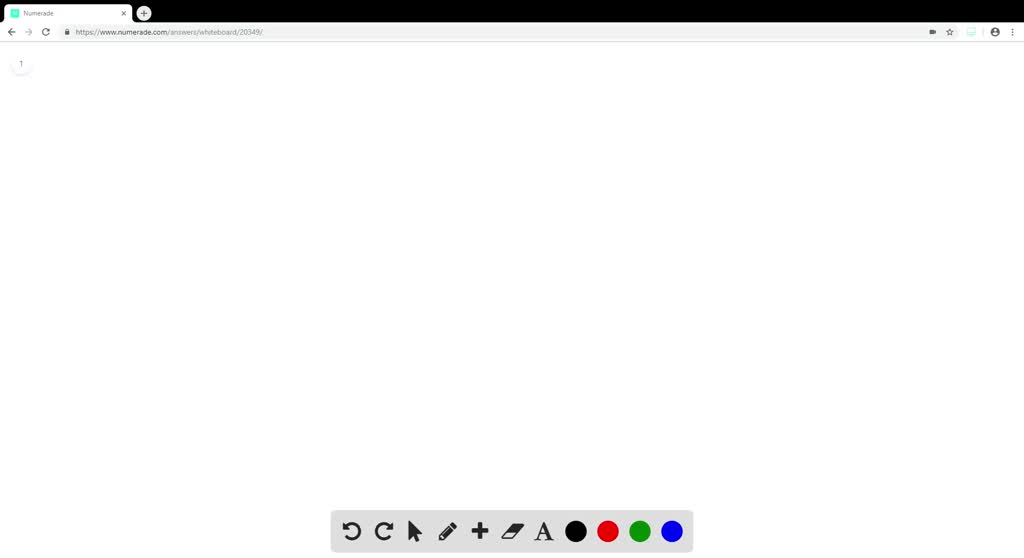This is a screenshot of the Numerade desktop website, showcasing its digital whiteboard feature. The overall background of the webpage is white, matching the whiteboard theme, while the website's top bar is black, providing a clear contrast. Below the top bar, there is a horizontally-arranged grey menu bar that houses various icons used for interaction with the whiteboard. 

The first icon is a circular arrow pointing left, representing the 'undo' function. Next to it is a circular arrow pointing right for the 'redo' function. A black cursor icon follows, allowing users to select objects on the whiteboard. There is also a pencil icon for drawing freehand, and a plus icon for adding images or screenshots. An eraser icon provides the functionality to erase content, and an 'A' icon enables text typing. Additionally, four color options—black, red, green, and blue—are available for drawing and text functions.